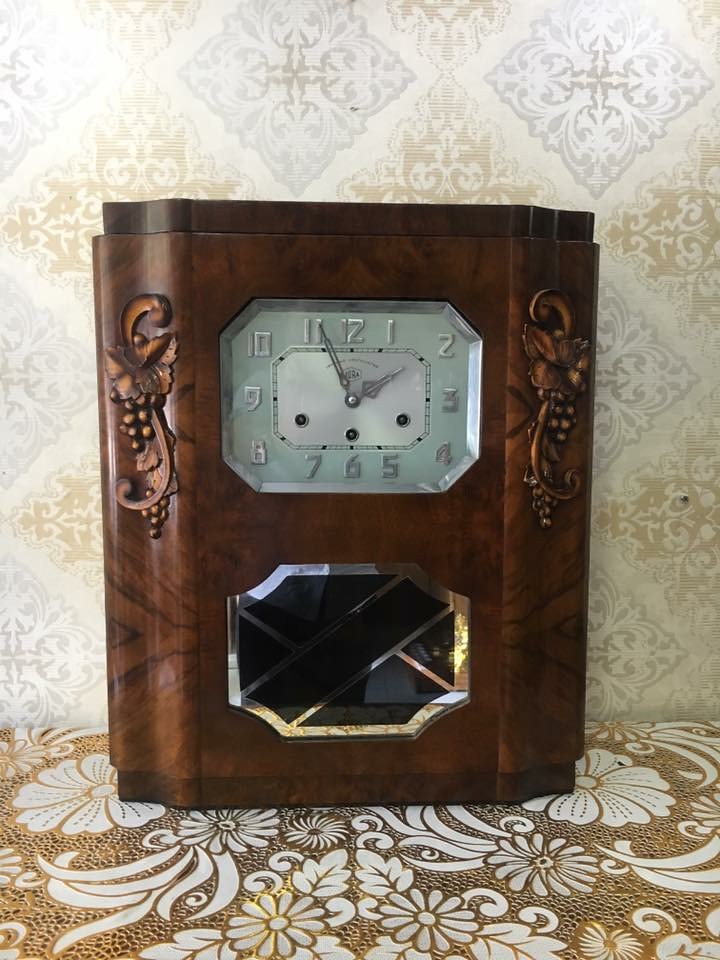The image features a vintage floor-standing clock housed in a wooden cabinet-like frame. The clock itself, positioned in the upper middle section of the cabinet, has a chrome finish and a unique flat, square shape akin to an elongated stop sign. The time displayed on the clock is five minutes to two. Below the clock face, at the bottom of the wooden frame, there is a similarly shaped glass panel framed in chrome, adding a cohesive aesthetic to the overall design.